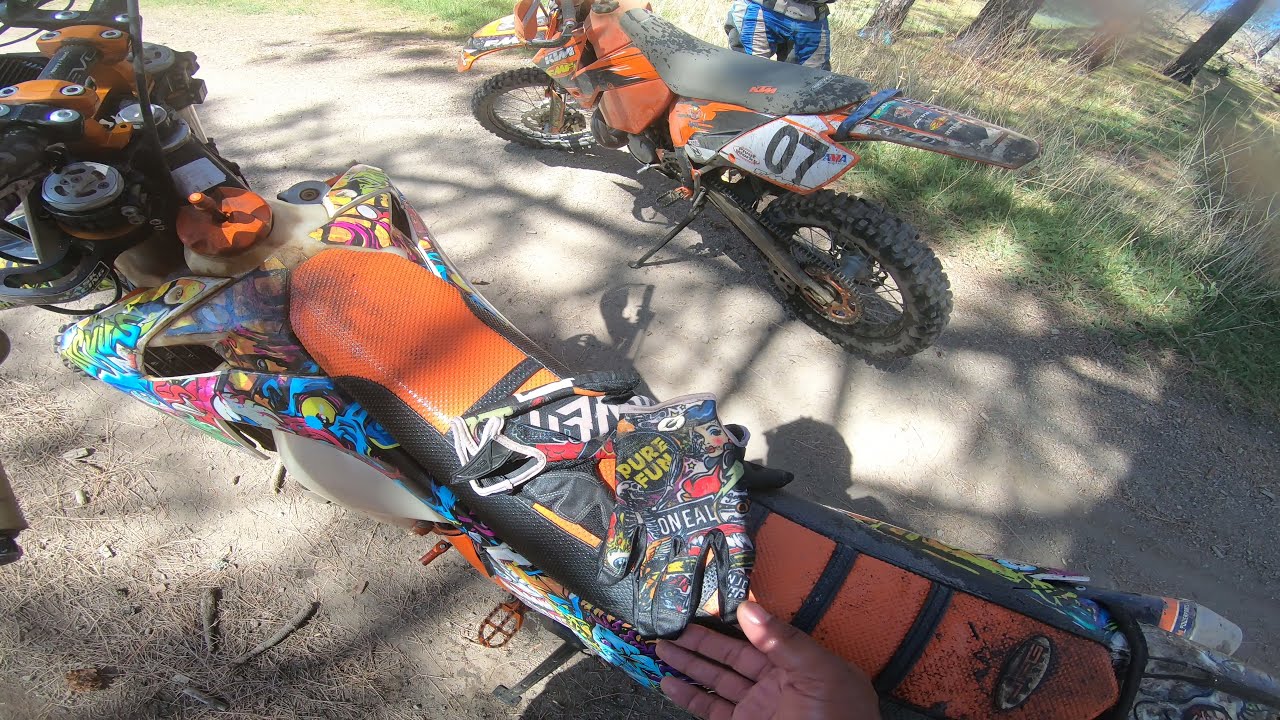In this detailed image, we are looking down on a group of dirt bikes positioned on a rugged dirt path strewn with branches, rocks, and compacted earth. The dirt bike prominently placed towards the center front is adorned with vibrant graffiti and splashes of blue, yellow, pink, and white colors. This bike features a distinctive orange seat accented with black lines and edges, with a unique pair of gloves resting on top. These gloves are covered in various graphics, including an illustration of a woman in a red dress with black hair. Adjacent to this bike is another dirt bike painted orange with a black seat and white trim, bearing the number 07 in bold black digits. Behind this numbered bike stands a rider dressed in a gray and blue suit. The scene is set on a dirt trail flanked by patches of grass and some trees in the distance, hinting at an outdoor, sunny day adventure.